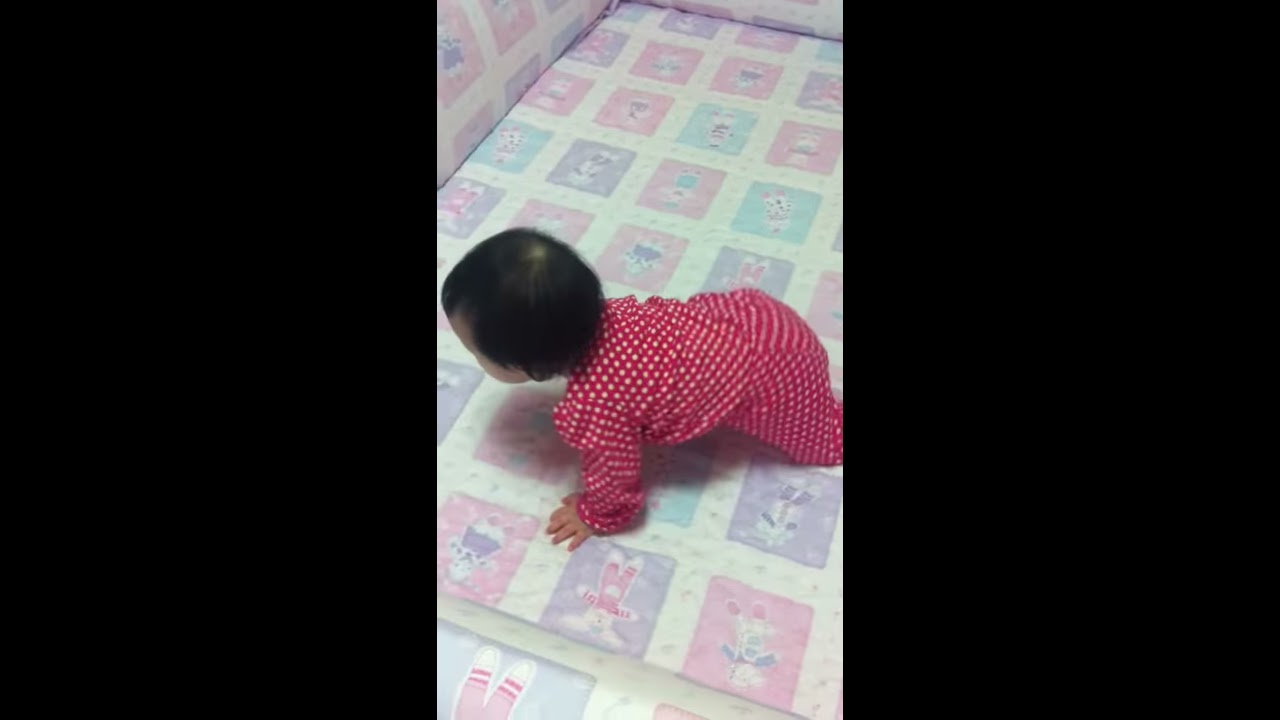In this detailed image, a baby, who appears to be a girl, is seen crawling on all fours. She wears a red onesie adorned with white polka dots that covers her arms and legs. Her dark brown, nearly black hair is short and thin, and a small bald spot is visible on the back of her head. The baby is crawling on what looks to be a quilted blanket or crib sheet that features a patchwork grid design composed of various colorful squares. These squares, colored in pink, purple, cream, yellow, green, and orange, showcase different cute cartoon characters, including rabbits and other small animals. The blanket or sheet extends over the bottom and up the side, suggesting it might be part of a crib or couch setup, and what seems to be a bumper pad is visible on the left side of the image. The scene is filled with soft, cushioned textures and playful patterns, creating a cozy and safe environment for the baby.